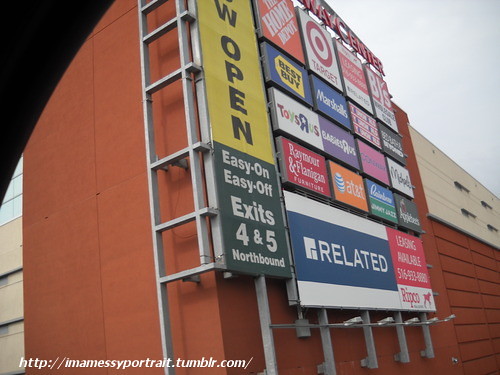This photograph captures a vibrant commercial building, taken from the perspective of a passing car's window, evidenced by the slight curve of the car window visible in the upper left corner. The building, constructed of orange brick, is adorned with a series of eye-catching signs, each promoting different businesses and services. 

Starting from the left, a vertical sign announces "Now Open" in bold black font against a yellow background. Below it, further details provide directional guidance with "Easy On, Easy Off, Exits 4 and 5, Northbound." The building continues to display an array of store logos, including The Home Depot, Target, BJ's, Best Buy, Marshalls, Toys R Us, and Babies R Us, interspersed with a few signs that are difficult to discern. An AT&T logo is also visible towards the bottom.

At the base of the signage, a prominent banner reads "Related, Leasing Available," followed by an indistinct phone number. The angle of the photo highlights the signs on the left, while those on the right gradually fade out of clear view. Adding a final touch, the bottom of the image features the URL "http://imamessyportrait.tumblr.com/."